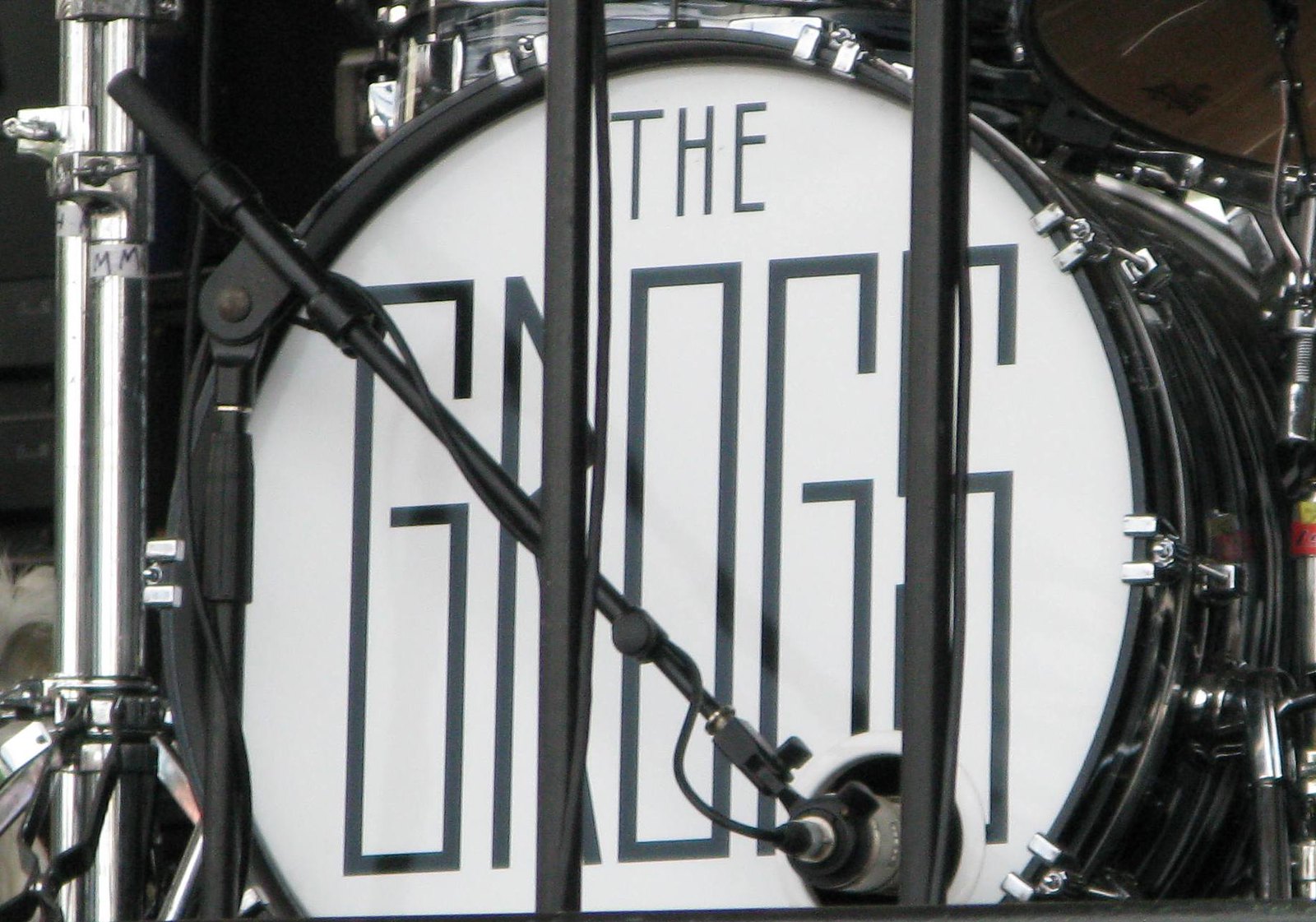The image features a close-up of a drum set, prominently displaying the front face of a bass drum. This bass drum is predominantly white with black letters spelling out "The Groggs," likely indicating the band's name. A microphone, positioned diagonally from its stand, protrudes towards the drum, capturing the sound from a hole in the drumhead. The scene is primarily rendered in black and white, with the metallic components of the drum set adding a sleek contrast. While the focus is on the bass drum, partial glimpses of other drum set elements are visible in the background.